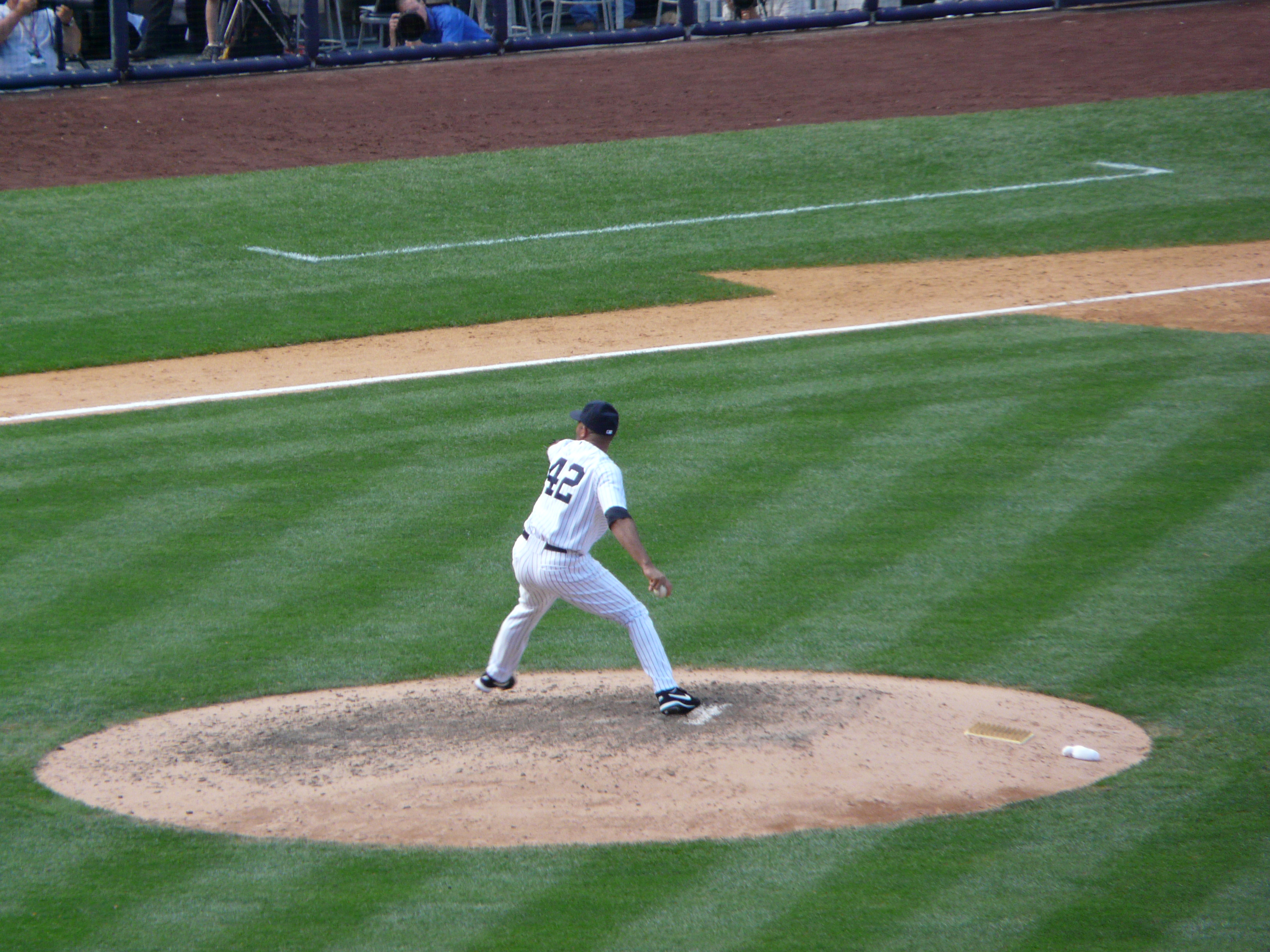In the image, Mariano Rivera, renowned pitcher for the New York Yankees, is captured mid-pitching motion on the mound. He is adorned in the Yankees' iconic white pinstripe uniform, with the number 42 emblazoned in blue on his back. Rivera's right foot is firmly planted on the pitcher's mound rubber, while his left foot is poised to step forward. The pitcher is in his distinctive black Yankees cap, pulling back his right arm, which holds the ball, ready to deliver a pitch. His legs are spread wide, showing his classic throwing stance. The scene is set in the distinct pitcher's circle of dirt, surrounded by the well-maintained green outfield and the neatly painted third baseline, indicating the runner's path. A glimpse of the dugout and its occupants can be seen, along with some photographers positioned behind the background wall, capturing the moment. Additionally, the rosin bag is visible on the side of the mound, adding to the authenticity of this in-game action shot.